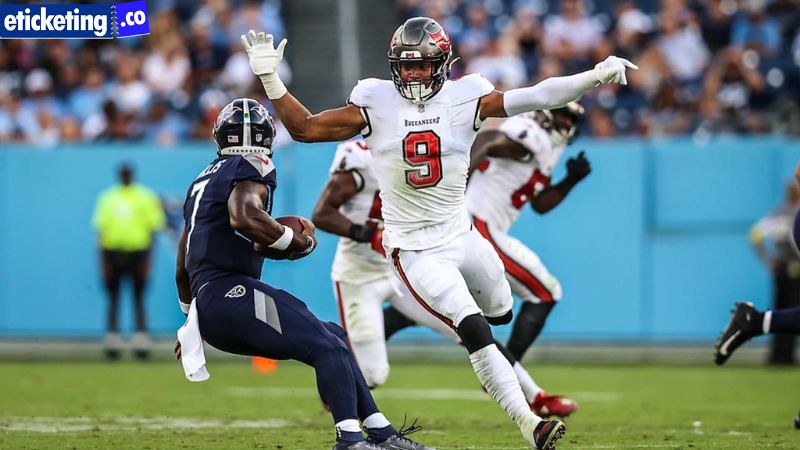The image captures an intense moment of a football game between the Tampa Bay Buccaneers and the Seattle Seahawks. In the foreground, a Buccaneers player clad in a white uniform with red lettering and a black helmet, identified by the number 9, is in a dynamic running pose with his right hand up and his left arm extended. He appears to be either attempting to block or reach out toward the Seahawks player. The Seahawks player, wearing a blue uniform with the number 7 and a black helmet, has just caught a pass and is poised to run, though his balance looks precarious, possibly due to his momentum. Behind these central figures are two additional players from the Buccaneers, mid-action but not focused on the immediate play. The grass field is vividly green, adding contrast to the colorful uniforms. The blurred background reveals a filled stadium, with indistinct audience members and a blue-walled stand. To the left side of the image, a referee or security person in fluorescent yellow is partially visible. Notably, the top left corner of the image features the text "e-ticketing.co" in white against a dark blue background, adding a modern touch to the scene.